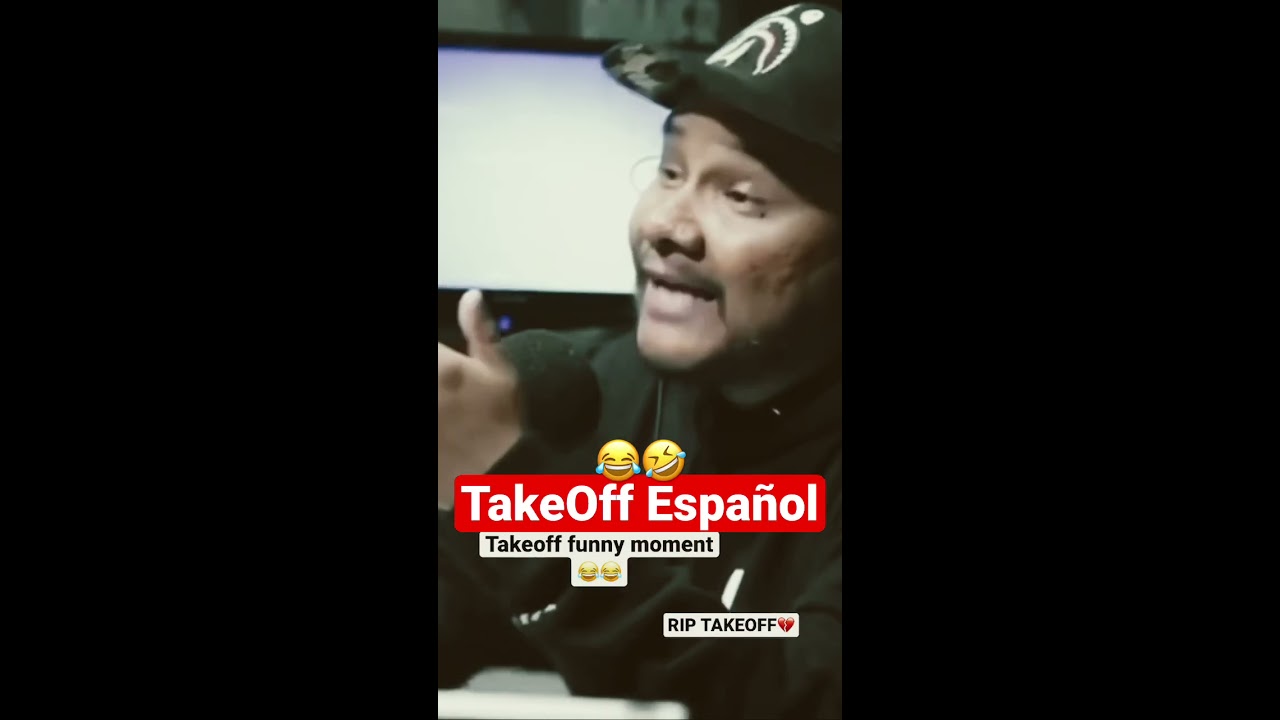The image appears to be a screenshot from a phone, showcasing a video with the vertical orientation typical of mobile recordings. Framed by large black rectangles on both sides, the central photo features a Hispanic man, likely in his 40s or 50s, who appears to be in mid-conversation. He is wearing a black baseball hat with white embroidery and a dark long-sleeved shirt, giving a glimpse of a computer monitor behind him. The man, who has a light mustache, is captured with his mouth open, possibly as he's talking or laughing, and raises one hand, which might be holding a microphone.

Text overlays are prominently displayed on the image. Directly over the man's chest, a red banner reads "Take Off Espanol," flanked by two laughing smiley emojis. Below it, a white banner says "Take Off Funny Moment," and includes two additional, indistinguishable icons. At the bottom, another white banner states "RIP Take Off," accompanied by a broken heart emoji. Various color elements such as black, white, red, yellow, blue, gray, and green can be seen, suggesting different elements in the background and the text overlays.

Captured in a lively and somber mix, this poignant moment is visually enriched with multiple emojis that tell a story of humor and loss. The man's expressive gesture and the textual elements portray a scene that is both engaging and pensive.